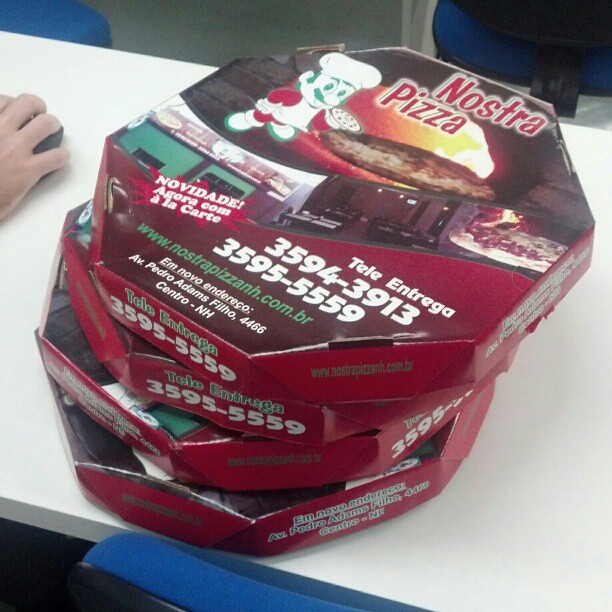In this indoor office setting, a white smooth table is surrounded by several blue-cushioned office chairs. One of the chairs is tucked in at the bottom left corner, while another is visible in the top left corner, and the backrest of a third chair can be seen in the top right corner. A person's right hand, possibly holding a computer mouse, is also discernible at the edge of the table. Dominating the center of the table is a stack of four octagonal pizza boxes from Nostra Pizza, each adorned with a red trim. The boxes feature imagery of a Mario-like chef character holding a pizza, with scenes of pizzas emerging from traditional flaming ovens and views of the restaurant's interior and exterior, which includes a green entrance. The text on the boxes includes phrases such as "Novidade, Agora con Alacarte" and "Teleentrega" with the contact numbers 3594-3913 and 3595-5559, along with the website www.nostrapizzanh.com.br. The address listed is M. Novo, Endereço Avenue, Pedro Adams Filho, 4466 Centro NH.